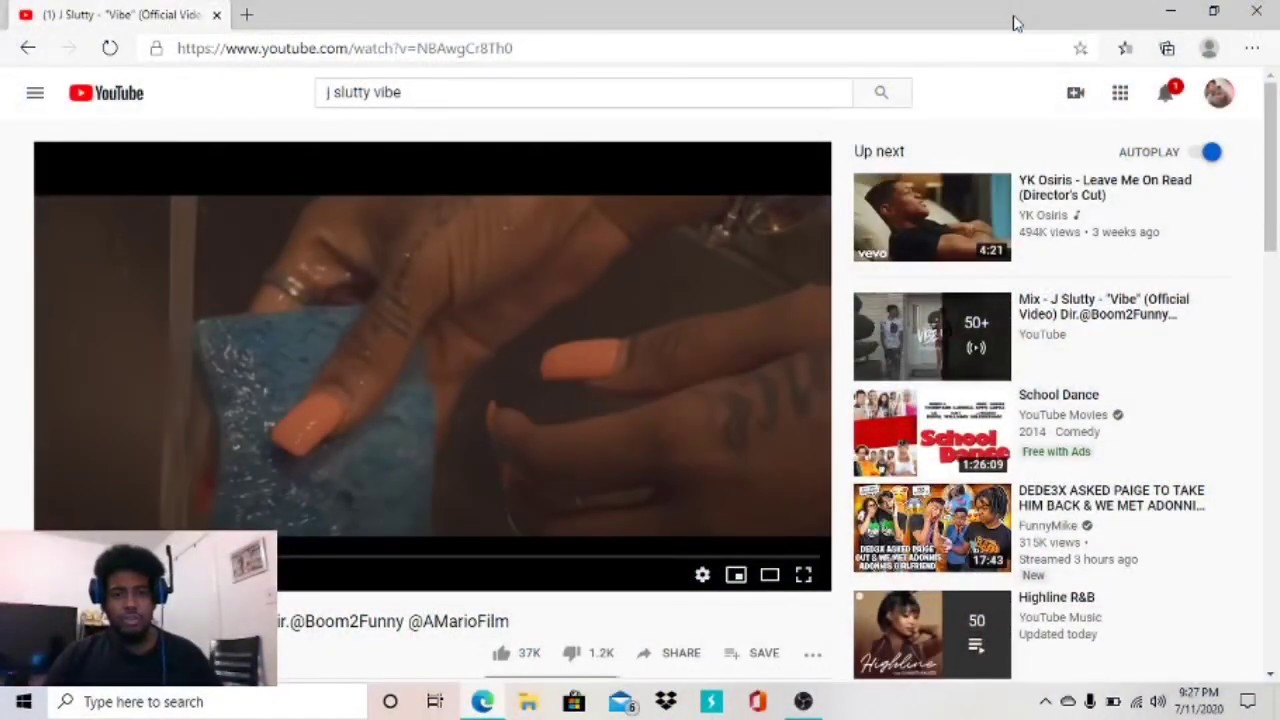This image is a screenshot of a web browser in landscape mode, captured on November 20, 2020, at 9:27 p.m. The upper left-hand corner of the browser window displays the search term "J. Slutty vibe." The background shows a list of various video thumbnails, including:

1. *Ys Osiris - Leave Me on Read (Director's Cut)*
2. *J. Slutty Vibe - Official Video (Directed by Boom Too Funny)*
3. *School Dance - YouTube Movies (Free with Ads)*
4. *DEDE 3x - Asked Page to Take Him Back and We Met Somebody*
5. *Highline - R&B (YouTube Music, updated today)*

The overall digital interface appears to be that of a familiar video streaming platform with a vertical scroll bar on the right-hand side.

In the bottom left-hand corner, there's an inset showing a person who is presumably watching the video. This individual is wearing headphones with the microphone lifted up and is positioned in an indoor setting. Behind them is a large monitor, indicating a possibly professional or dedicated work/study environment.

The bottom edge of the screenshot includes the typical display of an operating system’s taskbar, showcasing all open application icons. Additionally, the system time and date are visible in the bottom right-hand corner, reading "9:27 p.m." with the date "11/20/2020."